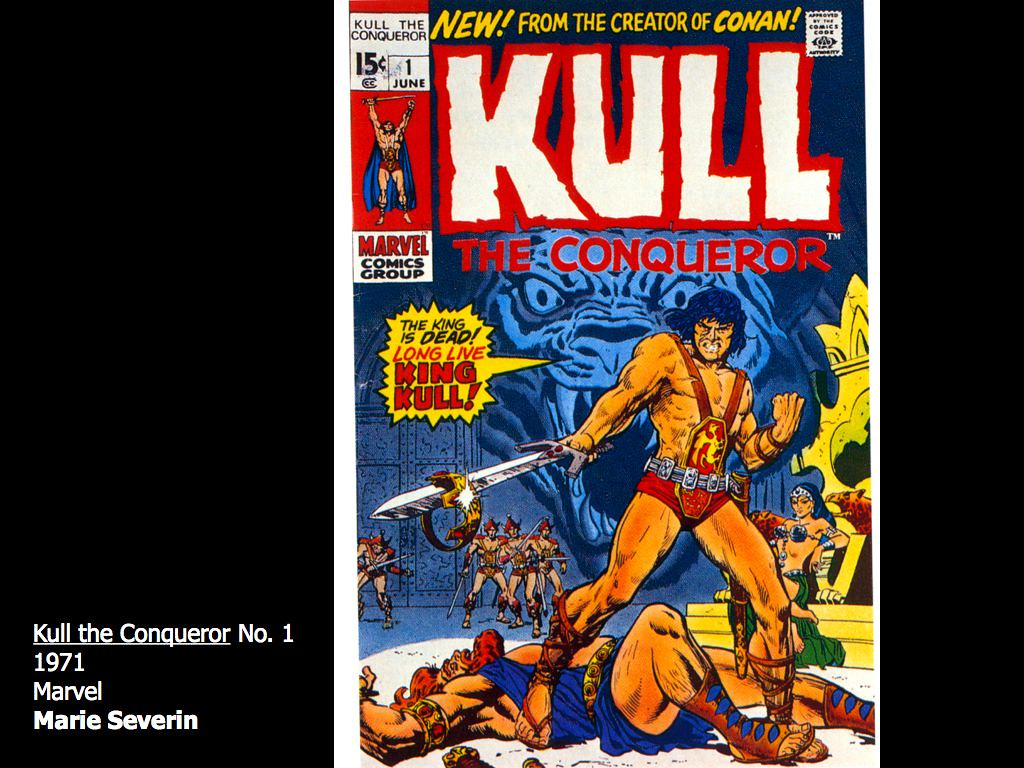The comic book cover image prominently features "Kull the Conqueror No.1" from 1971 by Marvel, illustrated by Marie Severin. At the top center of the cover, the text "New From the Creator of Conan" is displayed. The title "Kull the Conqueror" is boldly written just below this banner. On the left side of the image, there is a vertical black strip at the bottom of which additional credits read, "Marvel, Marie Severin."

In the artwork, a heavily muscled man is shown standing dominantly in an arena. He holds a sword in his right hand and wears a distinct red shield on his belly, secured by two red straps over his shoulders, resembling a red undergarment. This character stands over another man who is lying on the ground, dressed in blue cloth with red hair and a red beard, appearing lifeless. The scene is surrounded by other figures in the background, adding to the dramatic atmosphere of the illustration. On the right side of the cover, there is another smaller vertical black strip.